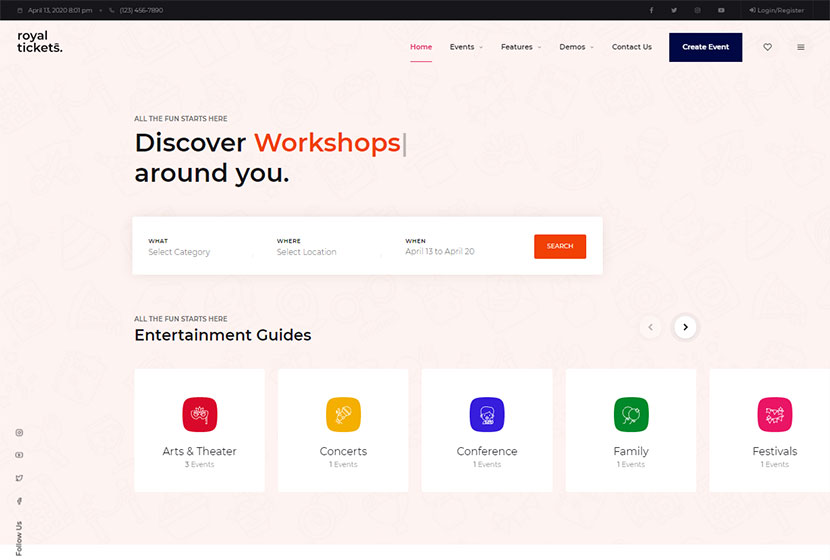The top edge of the webpage features a horizontal black rectangle that stretches across the entire width of the screen. On the left side of this rectangle, a small calendar icon is displayed, followed by the date and time "April 13th, 2020, 8:01 p.m.," in a very dark gray, almost illegible text. Accompanying this is additional text that is difficult to discern but appears to include a phone number.

On the right side of this black rectangle, the same dark gray text color is used for a series of social media icons: an 'F' representing Facebook, a bird silhouette for Twitter or X, an indeterminate logo, and a YouTube icon symbolized by a rectangle with a play button in its center. Further right, an unrecognizable symbol is followed by the text "login/register."

The background beneath this black rectangle transitions to a light pink. Positioned at the top-left of this section, the text "royal tickets." is written in all lowercase. On the top-right, several blue links are arranged in a horizontal sequence: "home," "events," "features," "demos," "contact us," and "create event." The "home" link stands out in pink, with a corresponding pink underline, while the "create event" link is distinctly highlighted in white and encased in a blue box. Adjacent to this array of links, a heart outline is visible, and further left of the heart, three horizontal lines stack vertically.

Beneath this navigation menu and located in the middle-left of the page, the text "ALL THE FUN STARTS HERE" is boldly written in capital, dark blue letters. Directly below, in a larger font with mixed capitalization, the phrase "Discover workshops around you." places emphasis on "workshops" by displaying it in orange.

A white horizontal rectangle stands prominently below this section, segmented into several fields: 
- On the left, "WHAT" is marked in bold, blue uppercase letters; beneath it lies the gray, slightly larger text "select category."
- The center section mirrors this format with "WHERE" in all caps blue, and "select location" in gray below.
- The rightmost section includes "WHEN" in the same blue uppercase letters, followed by "April 13 to April 20" in gray.

Completing this rectangle is an orange search button housing the word "SEARCH" in white uppercase.

Continuing down the page against the pink background, the phrase "ALL THE FUN STARTS HERE" appears again in blue, all-capital letters. Beneath this, in larger mixed-case font, "Entertainment guides" is also displayed in blue.

Five equally-sized white squares are aligned in a horizontal row below the guides text, each presenting a different logo and event category:
- The first square features a red logo with theater binoculars, labeled "Arts & Theater" in blue, followed by "3 events" in smaller text.
- The second shows a yellow logo with a white microphone for "Concerts" and notes "1 event."
- The third square possesses a blue logo with an indistinct image, titled "Conference," with "1 event" in smaller text.
- The fourth has a green logo depicting two people silhouettes, labeled "Family" with "1 event" below.
- The final box on the right contains a pink logo for "Festivals," though the central image is unclear, indicated by "1 event."

To the left of the fourth box, two small circles with blue arrow pointers—one pointing left and the other right—serve navigation functions; the left arrow is slightly faded, suggesting inactivity.

Lastly, along the very left edge of the page, vertical text facing left reads "FOLLOW US." Above this, four tiny logos for popular social media platforms (likely Facebook, Twitter, YouTube, and another unidentified platform) are lined up in corresponding order.